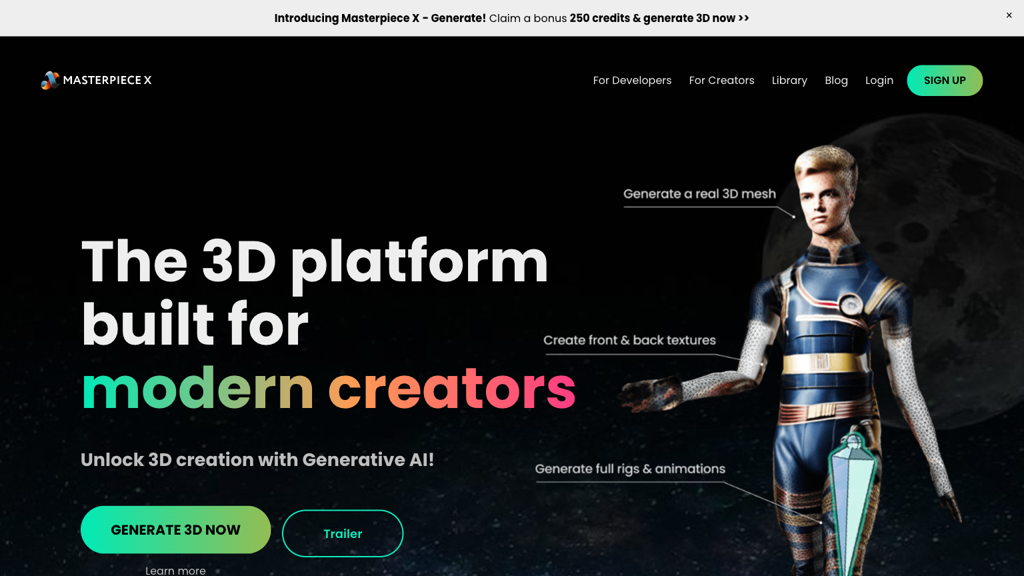### Website Home Page Screenshot Description

The screenshot showcases the homepage of a website with a light gray header at the top. In the center left of the header, bold black text reads "Introducing Masterpiece X-Generate!" followed by non-bolded text stating "Claim a Bonus." This is succeeded by bolded text proclaiming "250 Credits and Generate 3D Now!" with two black arrows pointing to the right. Towards the top right of the header, there is a medium gray 'X'.

Below the header, the main body of the page features a primarily black background. On the right side, there's a darkened image of Earth's moon, partly cut off by the edge of the frame, accompanied by a scattering of white and gray stars.

In the top left corner of the page, there's a colorful logo resembling a Mobius strip in blue, yellow, and orange hues. To the right of the logo, all-caps white text reads "Masterpiece X". A large expanse of negative space stretches to the right, leading to a menu with light gray text displaying the options: "for Developers," "for Creators," "Library," "Blog," and "Login." Next to the menu, there is a pill-shaped button with a gradient color transitioning from aqua blue on the left to greenish blue on the right, featuring black all-caps text that says "Sign Up".

Dominating the left side and extending to the screen's center, very large white text declares "the 3D Platform, Built For," with the phrase "Modern Creators" displayed on the third line in a gradient color ranging from aqua blue on the left, through pink in the middle, to orangish on the right.